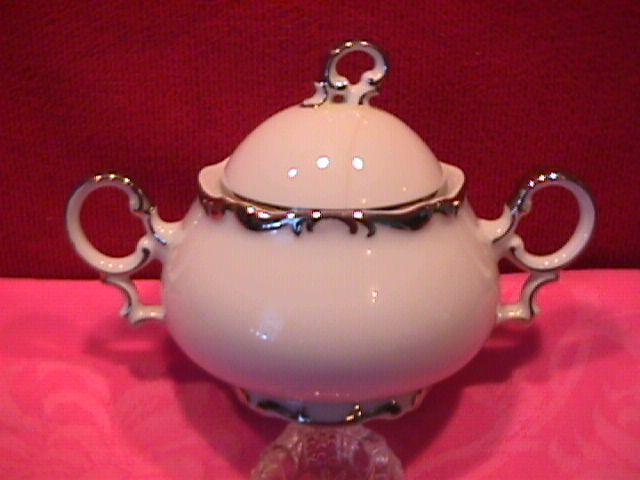This color photograph captures a single, centrally positioned China sugar bowl, prominently displayed against a backdrop of rich fabrics. The background is split into two sections: the upper area is crimson, while the lower area is pink, both adorned with intricate leaf-like designs. The bowl itself is a lustrous, milky white ceramic, which subtly reflects overhead lighting in soft white dots. Accented with gilded highlights, the sugar bowl features ear-shaped handles on either side, a small pedestal base, and a lid topped with a gold-rimmed loop handle. The harmonious blend of red, pink, white, black, and silver tones creates a visually striking and elegant image that could be seen in a store display, as a collectible, or as a meticulously wrapped gift.